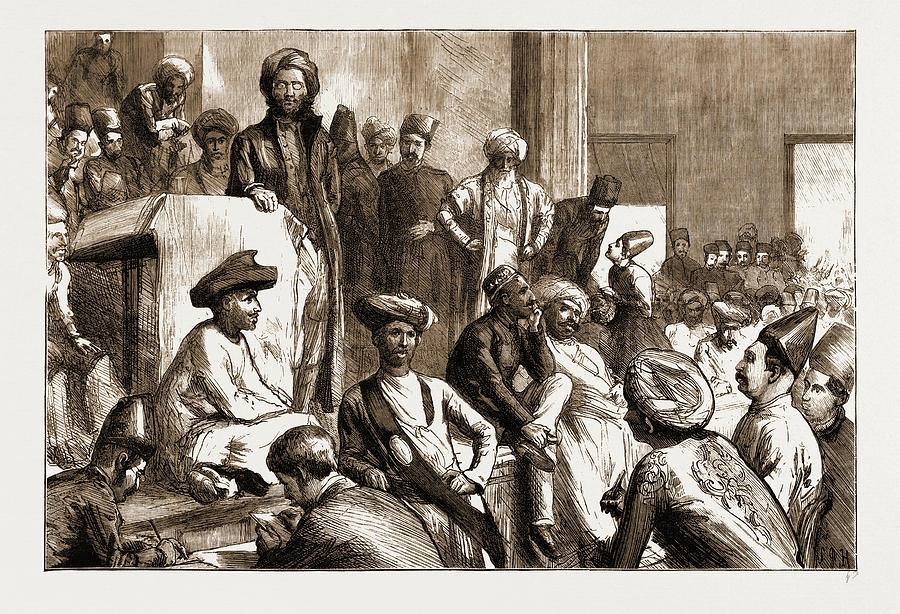The black and white illustration, titled "The Native Agitation in India, a Meeting in the Town Hall," depicts a detailed scene of a large gathering in a spacious hall with a high ceiling. The setting is divided into two tiers: a ground level where individuals are seated and a raised platform where others stand around a central podium. At the podium, located in the upper left-hand corner, a man stands with one hand on the surface, addressing the crowd. Several people, about 20 in total, are depicted throughout the image, both standing and sitting.

The attendees primarily appear to be from India, inferred from their attire. Many are adorned with headpieces, roughly divided between those wearing turbans and those wearing tall, straight hats. Notably, one individual in the front sports a hat that resembles a sailboat. Another figure crouches nearby, distinguishable without a hat and clothed in a Western suit, contrasting with the others who wear long coats, jackets, and robes.

To the right of the central figure at the podium stand two men, one in a dark robe with a turban and the other in a white robe. In the left corner, an officer-like character features prominently, identifiable by his large hat and white robe. The right-hand side of the image shows more seated individuals, only the tops of their heads and hats visible. The scene also includes architectural elements, such as a column in the center and a door at the back, adding to the depth and structure of the hall.